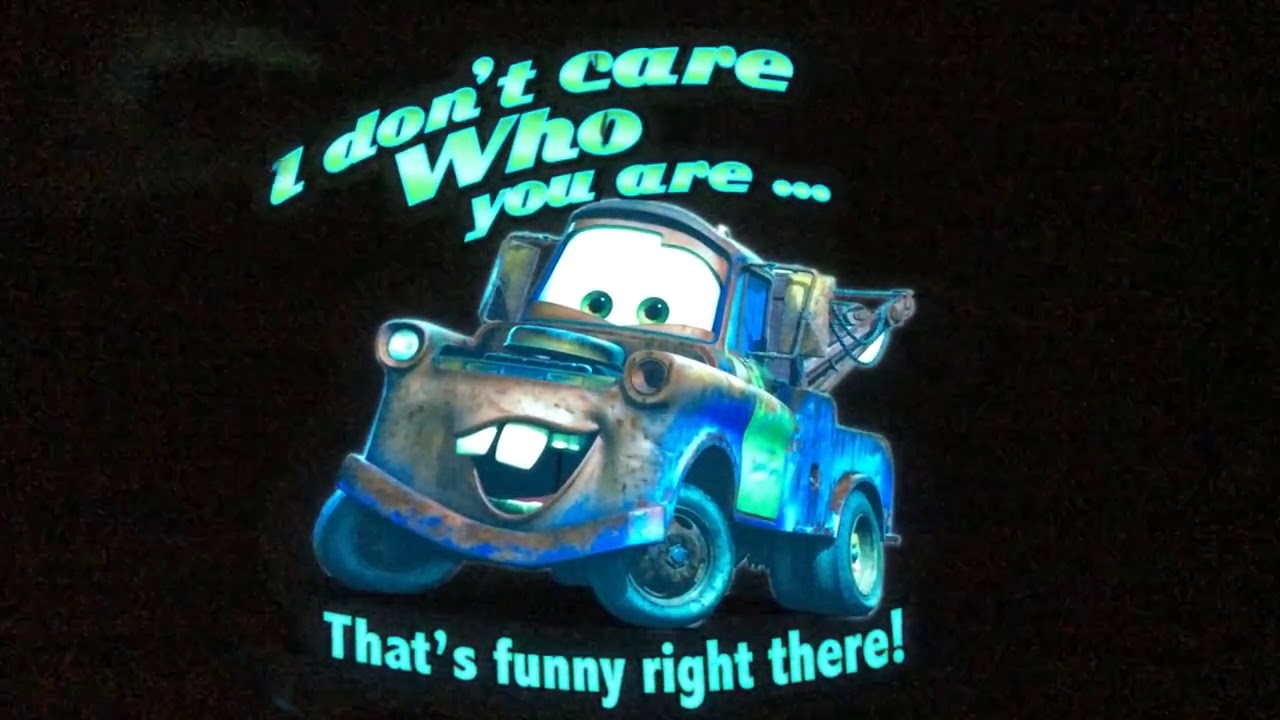The image features Tow Mater, a character from the Pixar movie *Cars*. The jovial, anthropomorphic tow truck is adorned with large green eyes and a wide, buck-toothed smile. Despite his rusty and old appearance, he is highlighted with a blue tint, making him visually stand out against a completely black background. The scene captures his playful expression perfectly. At the top of the image, green and neon blue text reads, "I don't care who you are..." followed by the bottom text, "That's funny right there!" The overall vibe resembles a fun, nostalgic piece of merchandise, like a t-shirt design.